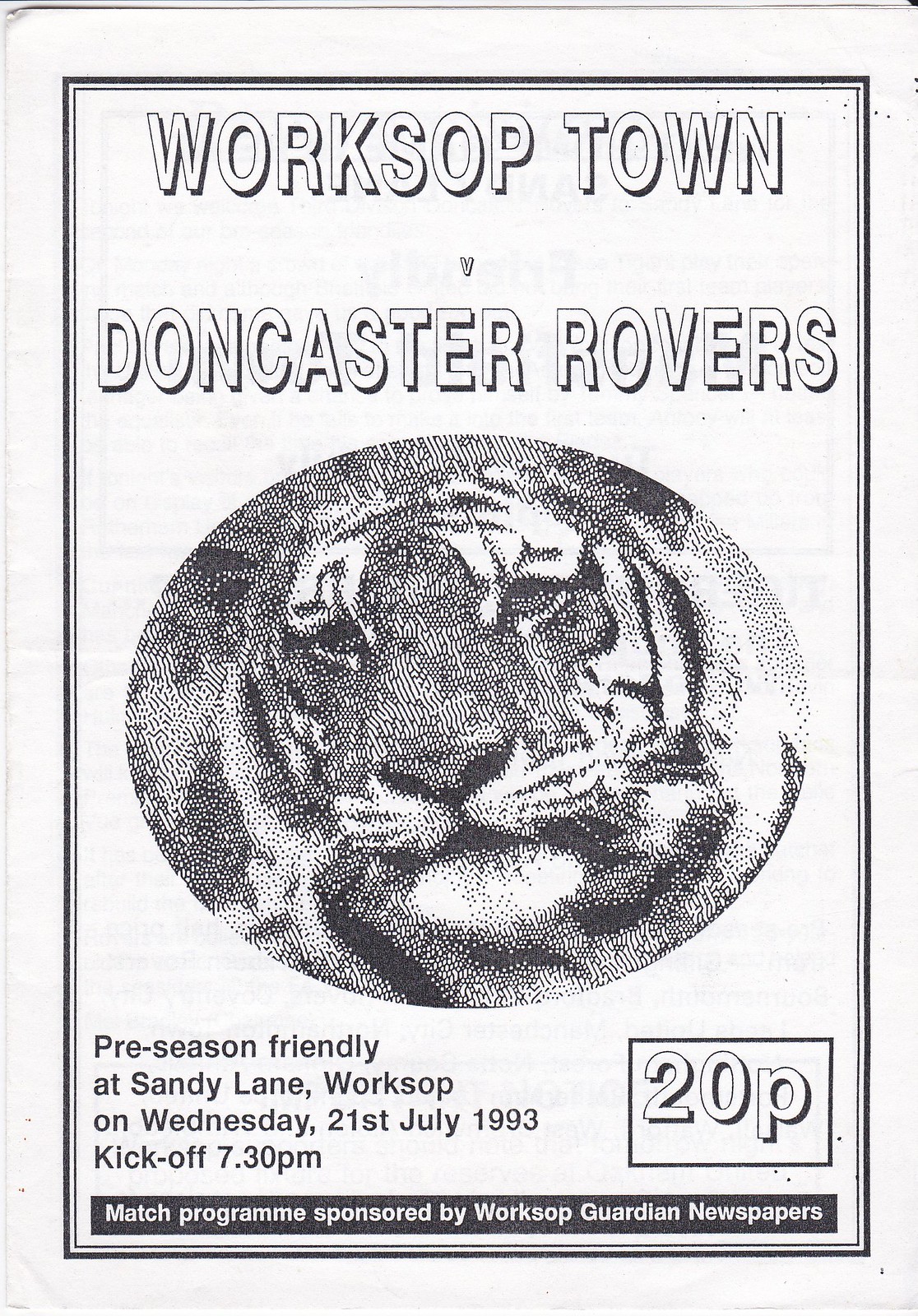This image is a black and white front page of a football match program for Worksop Town versus Doncaster Rovers. Dominating the center is a circular photo of a tiger's face, meticulously framed within the circle. At the top, bold text reads "Worksop Town, Doncaster Rovers." Toward the bottom, details of the event are clearly presented: "Pre-Season Friendly at Sandy Lane, Worksop on Wednesday 21st July 1993, kick off 7.30 p.m." The match program is sponsored by Worksop Guardian Newspapers. On the bottom right corner, there is a black-outline designating the price of "20p". The entire page is surrounded by a black frame, enhancing its black and white aesthetic.